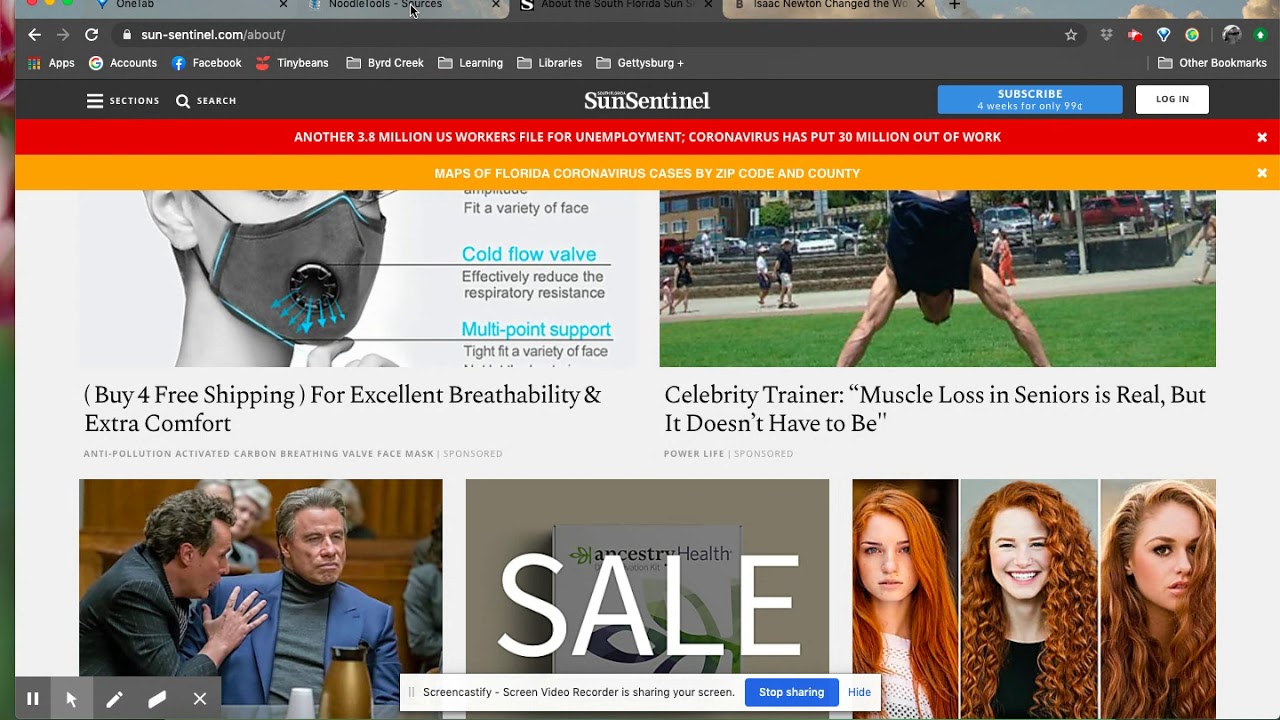The webpage from SunSentinel.com features a robust collection of news and advertisements. At the top of the page, viewers can see the newspaper's traditional font and logo, along with a prominent blue "Subscribe" button offering a subscription for 99 cents per week, and a "Login" option. Beneath that, a red banner highlights a significant news story: "Another 3.8 million US workers file for unemployment. Coronavirus has put 30 million out of work," accompanied by a subheading in orange detailing maps of Florida coronavirus cases by zip code and county.

On the left side of the page is an advertisement featuring a woman wearing a COVID-19 mask, touting features such as "excellent breathability," "extra comfort," a "cold flow valve," and "multi-point support to tightly fit a variety of faces." The ad emphasizes "buy four, free shipping."

To the right, an image of a celebrity trainer accompanies text discussing muscle loss in seniors: "Muscle loss in seniors is real, but it doesn't have to be." The trainer, a muscular man, is seen performing a handstand in what appears to be a park, with people visible in the background.

Further down is an image of John Travolta in a courtroom setting, dressed in a blue blazer, with a lawyer beside him, hand resting on Travolta’s shoulder. The middle section of the page highlights a sale for Ancestry Health, featuring a box of a DNA kit.

On the far right, an image of three young women in their twenties, all with reddish hair, potentially promoting a product related to makeup or hair dye, although no specific product details are mentioned. The women are diverse in their hair textures, with one having straight hair, another curly hair, and the third with a light brownish-blonde hue.

The page also includes navigation for different sections and a search bar at the top, completing the structured layout of this news web page.